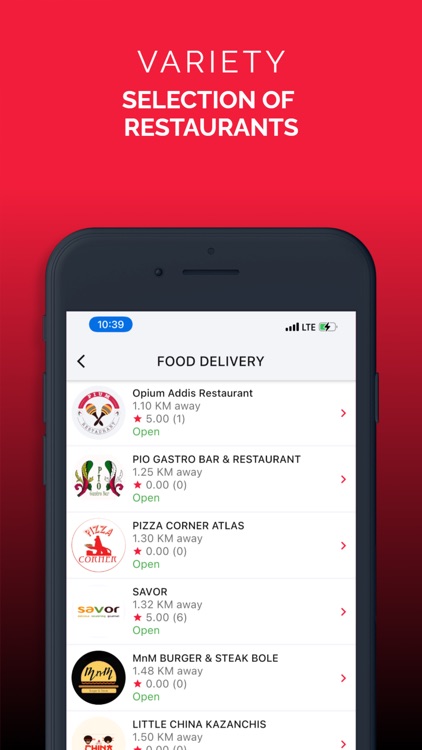In the image, a cell phone screen displays a search for "Selection of Restaurants" against a vibrant red background that gradually fades into maroon and then into a dark, light black hue towards the bottom. At the top of the image, the text "Selection of Restaurants" is prominently displayed in white. The cell phone screen lists several food delivery options, all within a 2-kilometer radius. The restaurants listed include:

1. **Opium Addis Restaurant** - Open
2. **Pio Gastro Bar and Restaurant** - Open
3. **Pizza Cornerapolis** - Open
4. **Savor** - Open
5. **M&M Burger and Steak Bowl** - Open
6. **Little China Kazan Cheese**

Each restaurant is accompanied by its emblem, represented in various colors, positioned on the left side of their respective listings.